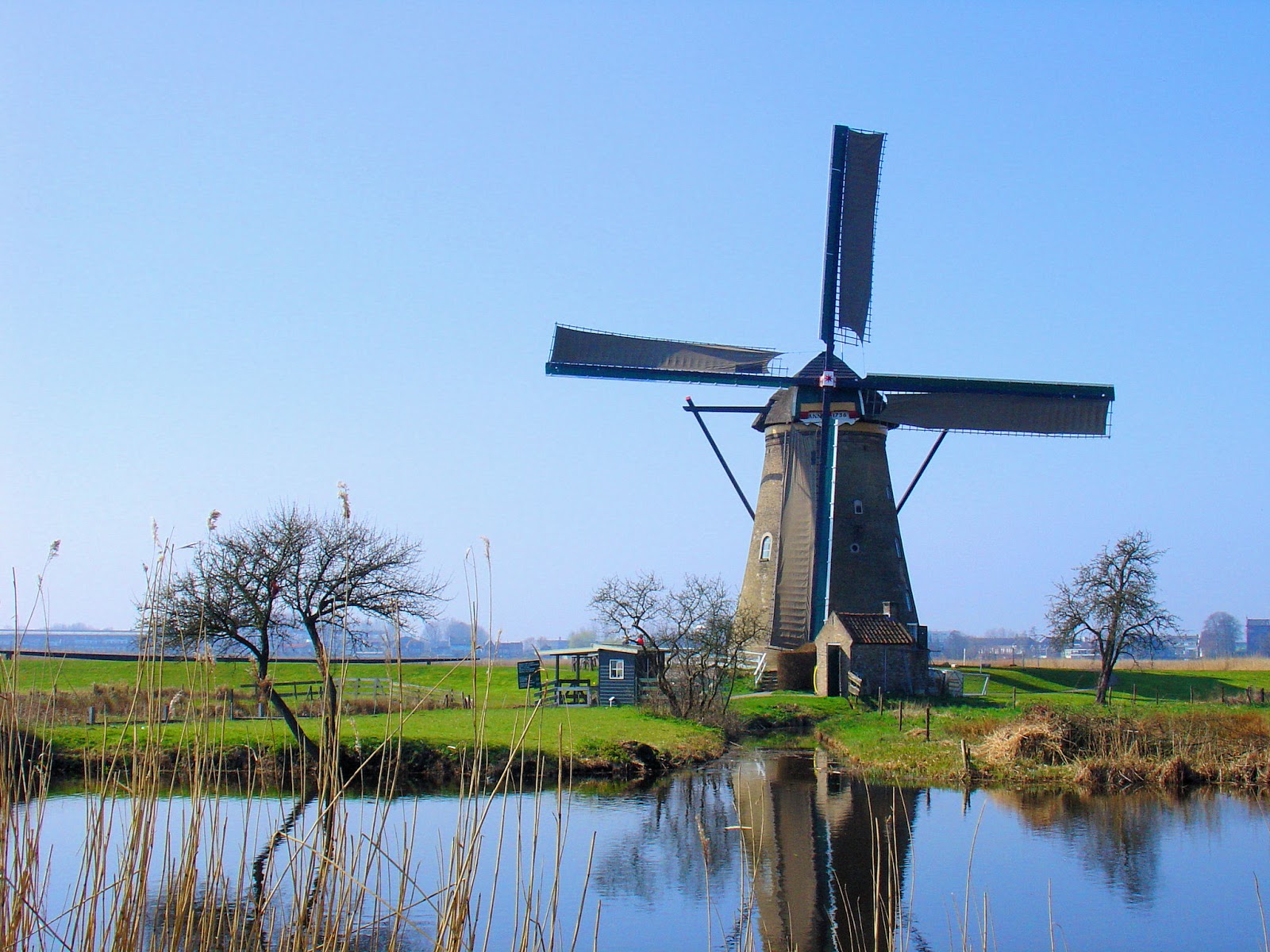This daylight outdoor photograph captures a picturesque scene possibly set in Holland, featuring a classic windmill at the center. The windmill, notable for its traditional design with a triangular top and a cylindrical gray body, has four blue sails, though some descriptions mistakenly mention three. In front of the windmill, and slightly to the left, stands a small farmhouse with a brown, triangular-tiled roof. To the right of the windmill, there's another small blue house with a contrasting white roof. Both structures are set on a lush, green lawn. The foreground reveals a pond edged with brown, dry reeds and branches. On the other side of the pond, vibrant green grass leads up to the buildings. Some sparse trees and bushes are scattered on both sides of the windmill. The distant background, reaching the horizon, subtly shows additional buildings or possibly a distant cityscape, beneath a clear, cloudless blue sky. The entire scene is tranquil, with no indication that the windmill is currently in motion.